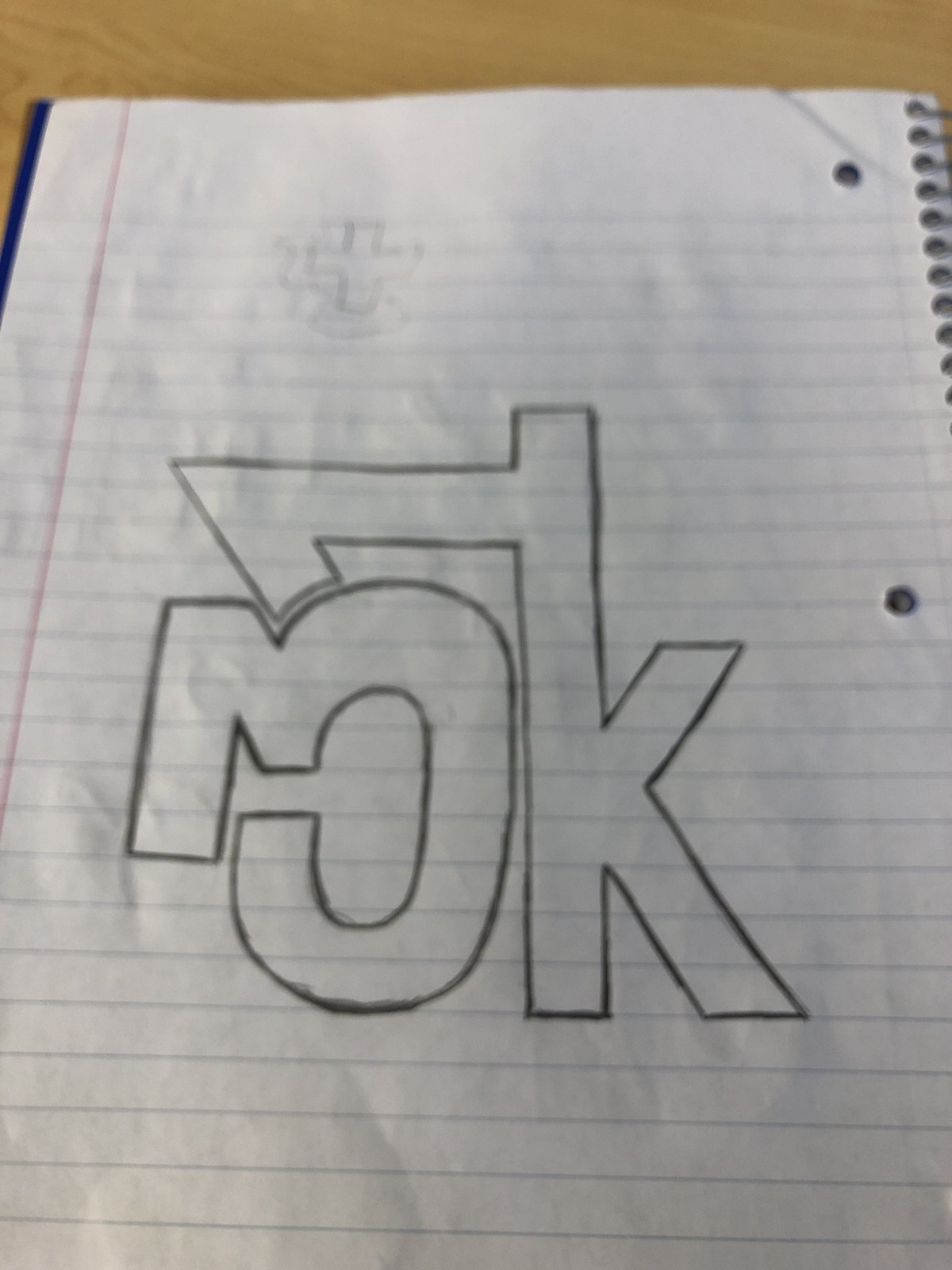This photo depicts a sketch on a page of white, lined notebook paper, taken from a spiral notebook with the spiral binding folded to the right side. The sketch consists of graffiti-style lettering that appears to form a backward lower-case "k" and a lower-case "c," with both letters intricately designed and connected. The "k" features a horizontal slash through its vertical stroke, while the "c" similarly has a small decorative element. Additionally, the drawing includes a faintly visible cross or plus sign in the upper left corner, accompanied by a small squiggle mark above it. The notebook is positioned on a light wooden table, suggesting a school environment. The paper shows signs of wear with slight wrinkles and visible punched holes, two clearly seen and the third partially visible. Overall, the drawing has a modernistic, logo-like appearance with a distinct, stylistic touch.